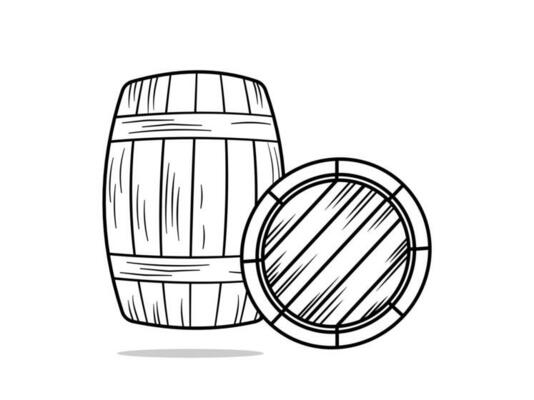In this black and white drawing, two wooden barrels are prominently featured against a translucent background. The barrel on the left side stands upright, casting a shadow beneath it that emphasizes its slightly levitating position. This barrel is composed of six vertical wooden slats, held together by two horizontal bands—one positioned a quarter of the way down from the top and another a quarter of the way up from the bottom. Adjacent and slightly overlapping this barrel on the right is another barrel that lies on its side, partially obstructing the view of the standing barrel. This horizontal barrel exposes its top, lined with six slats, and a securely fitted lid comprising eight sections, surrounded by a circular trim, is placed nearby. Both barrels are detailed with fine lines that accentuate their wooden texture, adding depth and realism to the simple, monochromatic illustration.